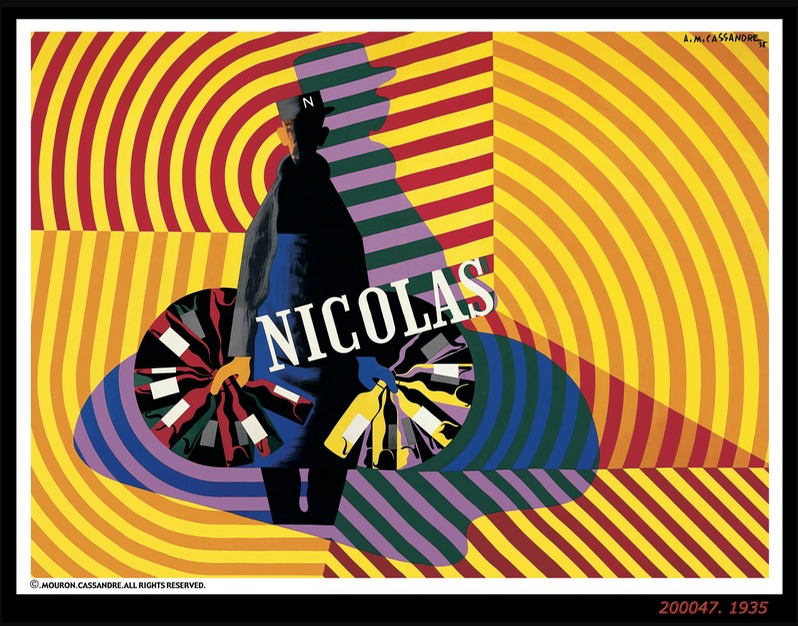This vibrant image, which could be a painting or a poster, bursts with color and intricate detail, illustrating a young man named Nicholas at its center. It features a background dominated by overlapping concentric circles and vertical stripes in various hues of orange, yellow, red, blue, green, purple, and dark tones. Nicholas, who has darker skin and his facial features obscured in shadow, is depicted wearing a hat emblazoned with the letter "N" and a dark jacket topped with what appears to be a blue dress-like garment over black pants. He stands with his arms extended, holding numerous wine bottles—red bottles in his right hand and yellow (white wine) bottles in his left hand, each bottle adorned with blank white labels. His stance and the positioning of the bottles give the impression that he is swinging them in a circular motion, contributing to the dynamic feel of the image. The word "NICHOLAS" is inscribed in white capital letters above him. The lower section of the artwork includes the artist's signature, "A.M.Cassandre," along with a logo featuring the letter "C" and the text "Moroch.Cassandre.All Rights Reserved." Additionally, within the white border that frames the image, the bottom right corner reveals the numbers "200047.1935."